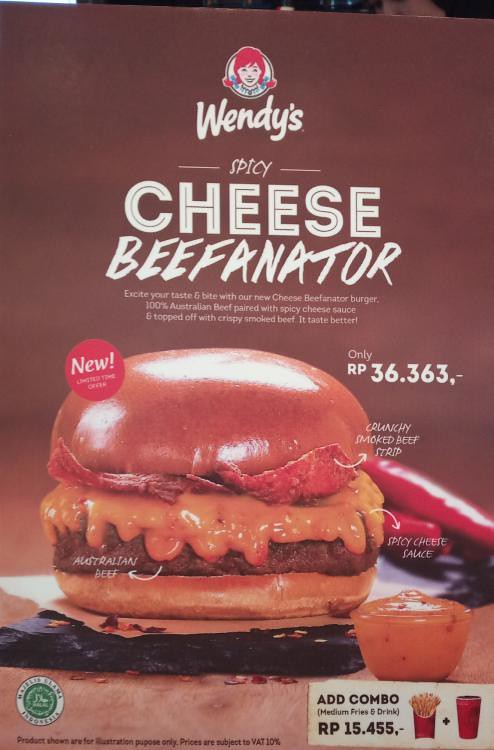Here's the cleaned-up and detailed caption:

---
This vibrant Wendy's advertisement showcases the iconic Wendy herself at the top center, with her unmistakable red hair styled in pigtails, and her blue dress with matching ribbons. Beneath her cheerful image, the Wendy's logo appears in bold white lettering. The focus of the ad is on the new Spicy Cheese Beefinator, introduced in emphatic capital letters, framed by a neat line on each side. Below, a mouth-watering description invites customers to "Excite your taste and bite with our new Cheese Beefinator burger," made with 100% Australian beef, paired with spicy cheese sauce, and generously topped with crispy smoked beef. 

In the center of the ad, a tantalizing image of the burger is displayed, heavily laden with cheese, almost to the point of overshadowing the succulent beef itself. The ad mentions a price of $36.36, presumably in Australian dollars, reflecting the premium quality of the ingredients. Additionally, customers can add a combo of medium fries and drinks for an extra RP 15.45. A green logo at the bottom signifies that this particular advertisement is targeted towards the Indonesian market.